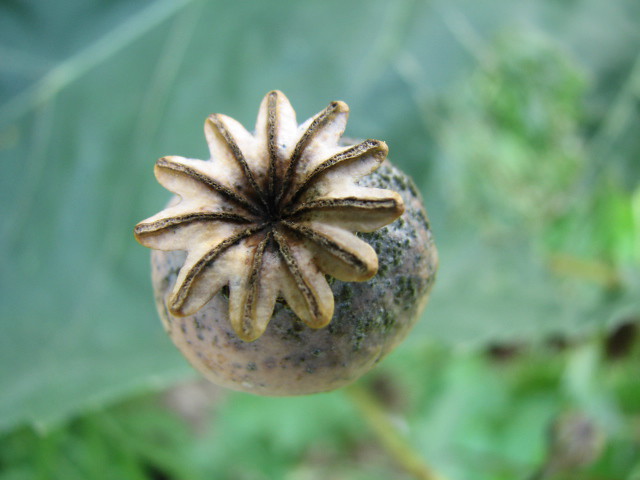This image showcases an extreme close-up of a plant, likely a poppy. The background is heavily blurred, providing a soft green backdrop composed of large leaves and foliage. The focal point is a prominent central stalk, crowned by a distinctive, round seed pod. Atop this pod, there's a unique, star-like structure with eleven pointed arms, resembling a starfish. The detailed textures and intricate design suggest that this is indeed the upper part of a poppy plant, often associated with the production of opium.